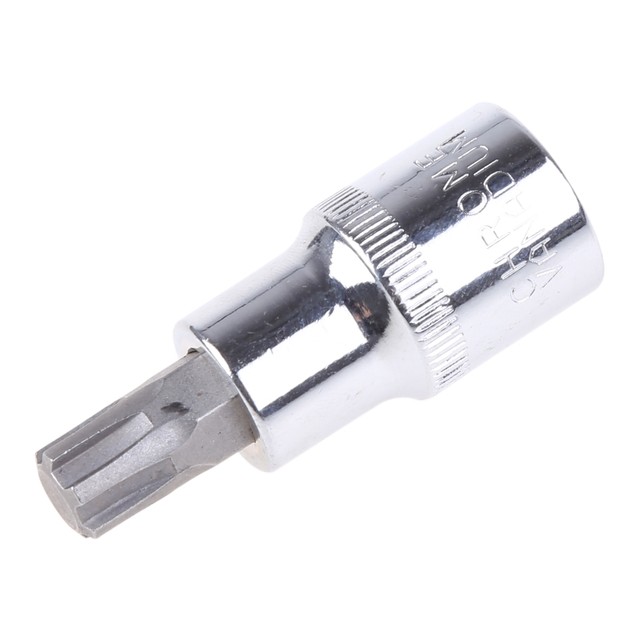This image captures a detailed, close-up view of a silver-colored socket driver for a power drill, set against a white background. The driver is positioned at a diagonal angle, running from the top right to the bottom left. On the left-hand side of the image, the bit's attachment end is clearly visible, featuring a dull, metal peg-type design with several teeth for secure latching onto a power drill. The upper right portion of the driver is seated inside a bright, polished, and shiny socket. The socket itself tapers from a thinner section to a wider base, where the words "CHROME VANADIUM" are etched prominently into the metallic surface. The tool's barrel displays a reflective, shiny metallic silver finish, contrasting with the tip's matte, unpolished appearance. A small black speck can also be seen on the tip, adding to the descriptive detail.